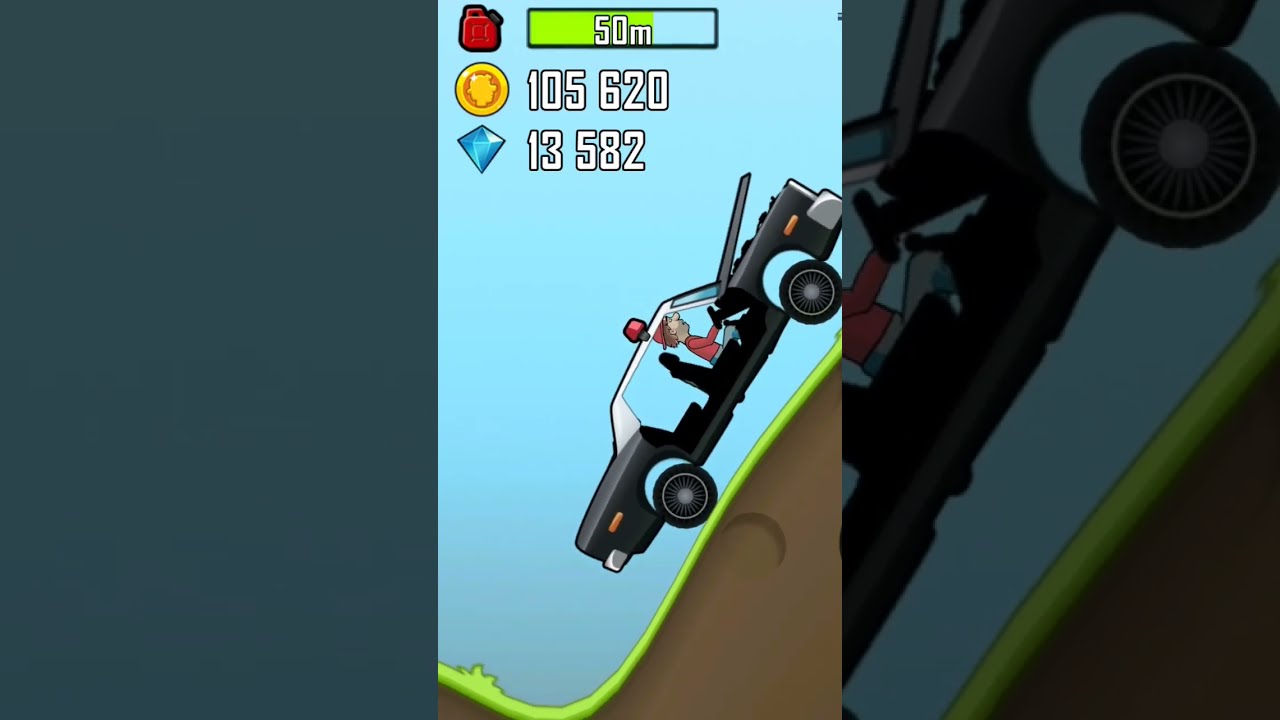The image is a detailed screenshot from a video game, likely designed for a smartphone. The scene centers around a man in a red shirt and red hat with a graying beard, driving an old, doorless, black-and-white police car with an active red siren. The car is tilted at a 30-degree angle as it ascends a grassy hill with brown dirt under a blue sky. Positioned slightly off-center to the right, the car is the focal point of the image. Above the car, in the top left corner, are various game icons and their respective metrics: a red gas can labeled "50M," a gold coin marked with "105,620," and a blue diamond with "13,582". The colors and design elements give the impression of a vibrant, engaging mobile game interface.